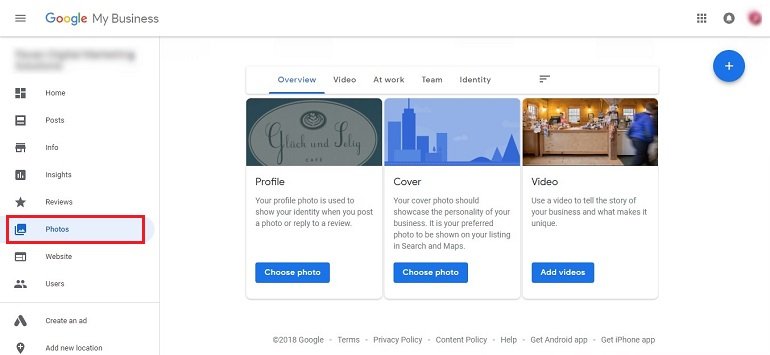The image is a detailed screenshot of the Google My Business interface on someone's Google account. 

At the top of the interface, the menu bar is present, starting with three horizontal lines on the far left, which provide more options when clicked. Next to these lines is the Google logo, followed by "My Business" in gray font. On the far right side of the menu bar, three icons are visible: a grid of nine dots representing different Google tabs, a gray circle with a white bell symbolizing notifications, and a slightly blurred circular profile picture of the user.

Below the top menu bar, on the left-hand side, there is a vertical column. At the very top, some blurred information, likely the user's name or personal details, is visible. This is followed by a list of sections that the user can navigate to, each with an icon on the left and the corresponding name on the right. The sections available are: Home, Posts, Info, Insights, Reviews, Photos (highlighted in blue indicating the current section), Website, Users, Create an Ad, and Add a New Location. The highlighted Photos section also has a red rectangle around it, indicating it might be part of a tutorial or suggested navigation.

Moving to the central part of the image, there is a horizontal menu displaying options such as Overview, Video, Work, Team, and Identity. The Overview section is currently selected. Below this menu, the interface splits into three columns. Each column offers different media-related choices, including the selection of a profile photo, cover photo, and the ability to add videos. Each option features a small cover image at the top, with corresponding descriptions in the middle. 

Overall, the layout is structured and provides a comprehensive overview of various management options available within Google My Business, with specific emphasis on the Photos section.